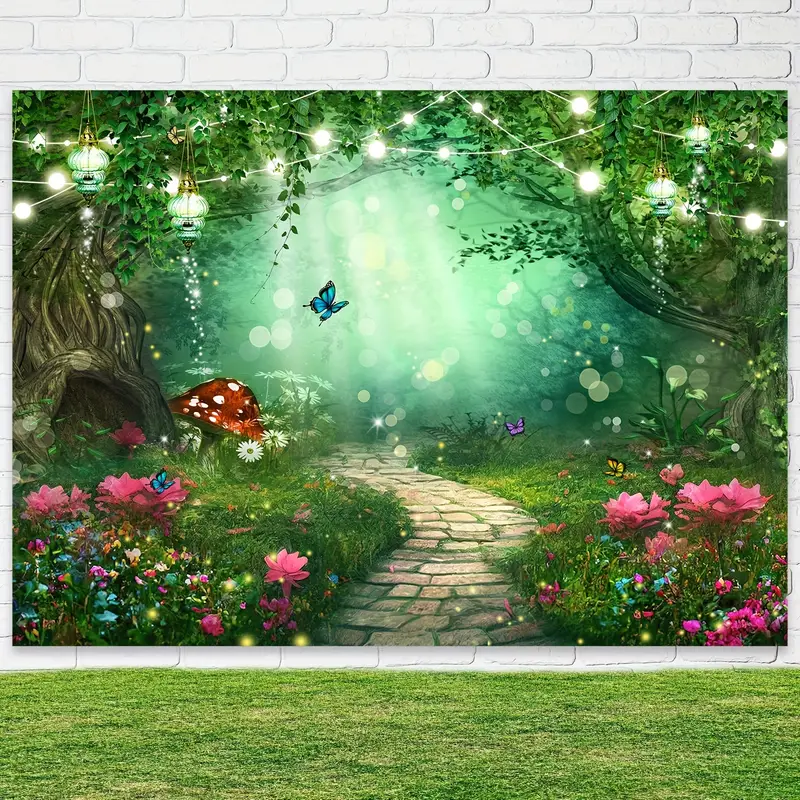The image resembles a high-resolution, computer-generated painting that captures a fantasy environment reminiscent of Alice in Wonderland. Set against a background of soft gray-white brick, possibly suggesting a mural, the scene is lush with vibrant green grass covering the ground. A stone pathway, with hints of grass sprouting between the stones, meanders through the scene. The pathway is flanked by vividly colored flowers in shades of pink, blue, and yellow. 

On the left, a whimsical tree trunk features a tunnel-like hole at its base beside a brown mushroom dotted with white spots. A butterfly, painted in striking blue, flits above the greenery. The top of the image features leaves and twinkling lights, mimicking sunbeams, creating a magical, fairytale-like ambiance. Sparkling lights and colorful orbs add to the enchanted feel of the scene. A cement divider lines the path, adding a subtle structural element amidst the natural surroundings. 

Overall, the image presents a captivating mix of natural and fantastical elements, meticulously detailed and vividly portrayed, making it a striking piece of digital art.